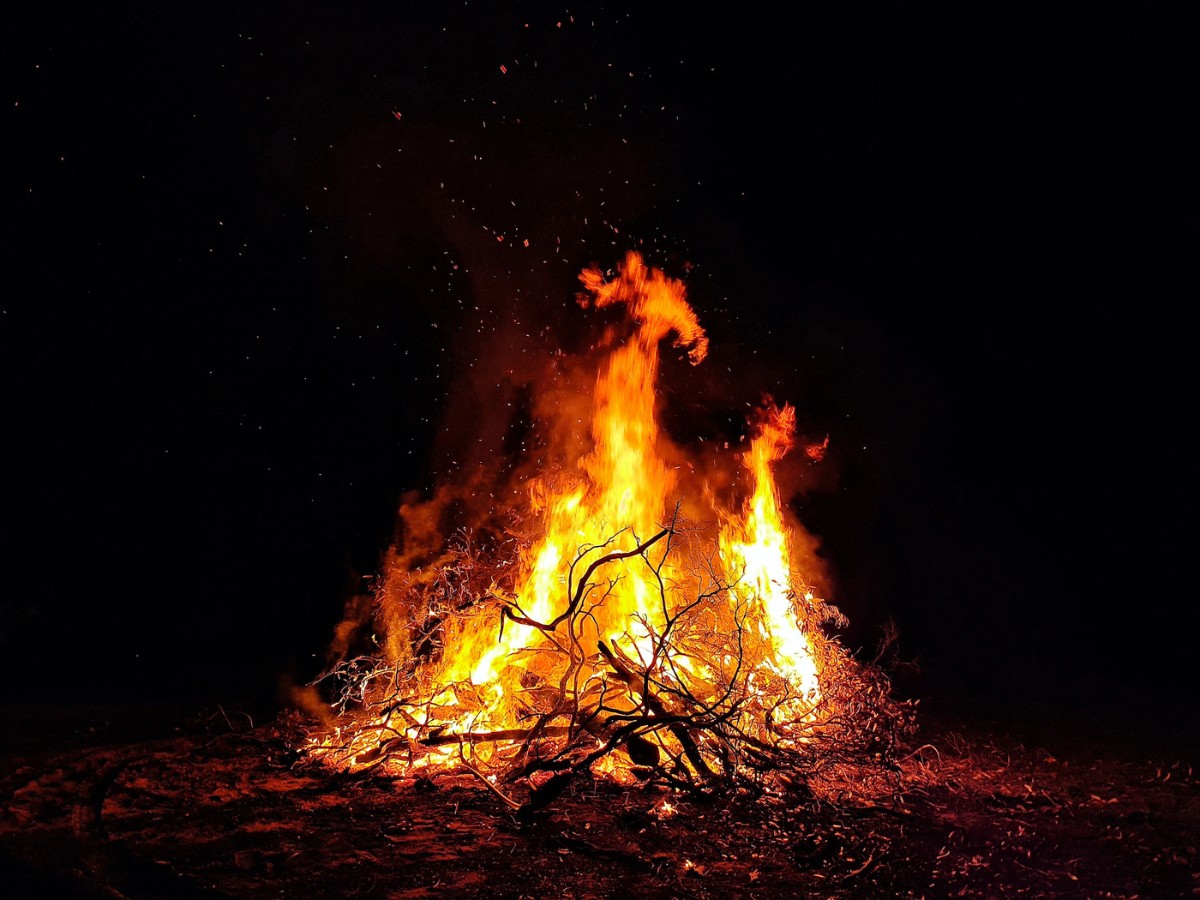The rectangular image, wider than it is tall, captures a vivid scene of a controlled bonfire in an otherwise pitch-black night. Dominating the center is the brightly lit campfire, composed of many logs and branches stacked high. The flames exhibit a spectrum of vibrant hues: the base of the fire glows an intense bright yellow and white, transitioning to deep orange in the middle, and culminating in striking reds and ambers toward the top. Occasionally, sparks and embers can be seen, their red and orange trails flying upwards against the unseen sky. The fire casts a warm, orangish-red glow on the nearby twigs, leaves, and foliage scattered on the ground in front of it. The ground, while mostly clear, shows small pieces of branches and foliage. Smoke billows gently to the left, and throughout the image, various shades of orange and amber from the fire illuminate the scene, highlighting the stark contrast with the surrounding darkness.